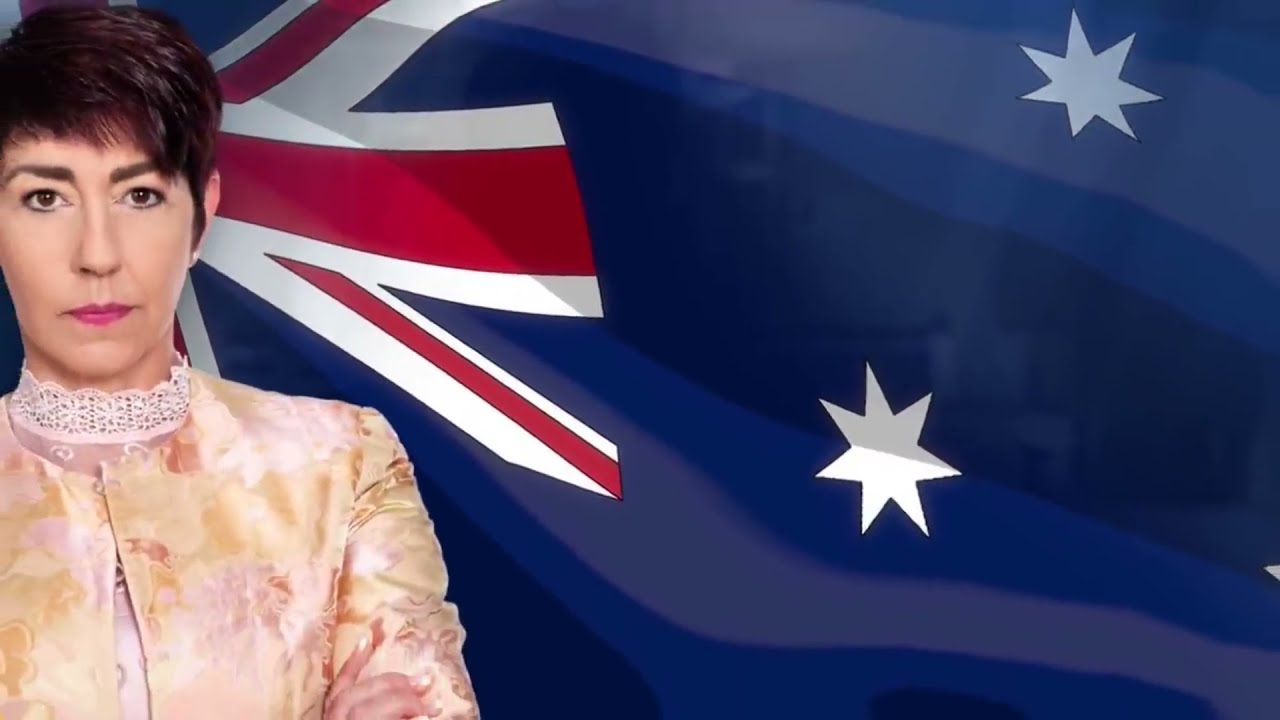The image features a stern-looking woman, possibly in her early to mid-40s, positioned on the left side, occupying approximately 30% of the frame. She has short brown hair and is wearing reddish-pink lipstick. The woman is dressed in a lacy blouse under a silky, pastel peach-colored button-down top. The combination of her attire and the stern look on her face gives a serious impression. 

In the background, taking up most of the right side of the image, is a close-up depiction of a flag suggestive of the British or Australian flag, in a waving motion. The flag features distinctive red, white, and blue colors with several blue stripes that squiggle slightly rather than being perfectly straight. There are also two seven-pointed white stars prominently placed within the pattern. The upper corner to the woman's left is highlighted by ribbons of red and white, adding to the intricate detailing of the flag backdrop.